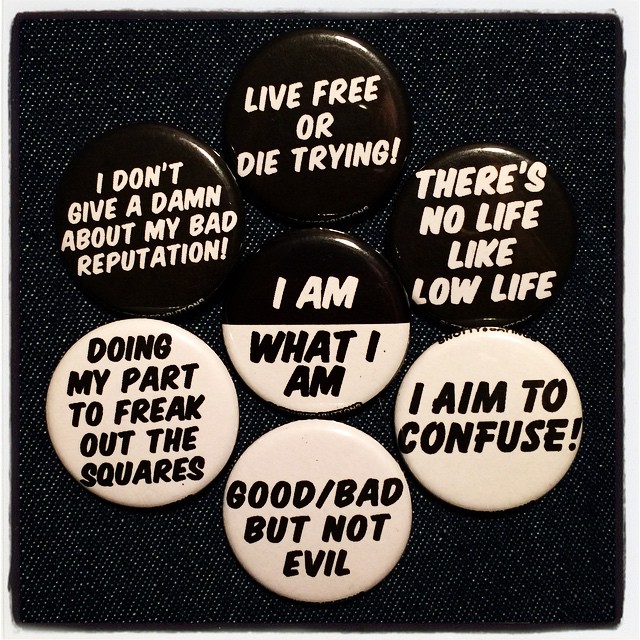This detailed photo features an artfully arranged collection of seven pin buttons displayed on a black fabric background. The buttons, circular in shape and varying in color scheme, are meticulously organized to form a flower-like pattern: three at the top, three at the bottom, and one in the center. 

At the top of the arrangement, the black buttons with white text declare, from left to right: “I don’t give a damn about my bad reputation,” “Live free or die trying,” and “There’s no life like low life.” The bottom row of white buttons with black text state, from left to right: “Doing my part to freak out the squares,” “Good/bad but not evil,” and “I aim to confuse.” The central button is uniquely designed with a black top half and white bottom half featuring alternating text colors, reading “I am what I am.”

The black fabric background, likely a piece of black jeans cloth, boasts tiny white speckles scattered throughout, adding an intricate texture to the setting. This organized and deliberate arrangement creates a visually balanced and cohesive display, ensuring that each button and its rebellious message is clearly visible and easily readable.